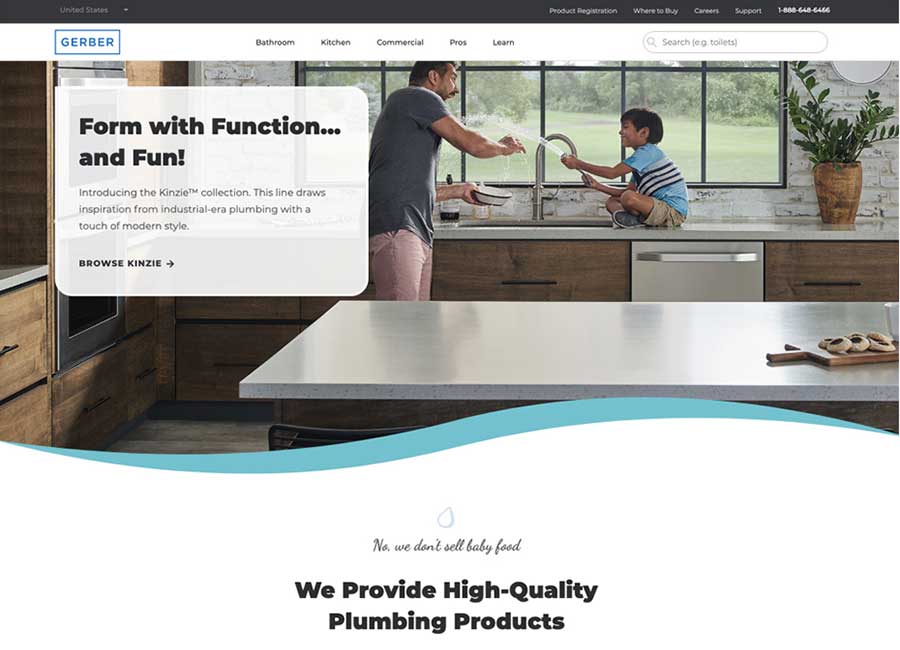The image on the computer screen displays a webpage for a company named Gerber, known for their high-quality plumbing products, not baby food. The majority of the webpage is occupied by a vibrant photograph capturing a lively kitchen scene. 

In the background of the photograph, there's a window offering a view of the outdoors. Central to the image is a kitchen sink with a sleek faucet. Standing to the left of the sink is a man holding a bowl in his left hand, and using his right hand to shield himself from a playful burst of water. The source of this water is a boy positioned on the countertop to the right of the sink, actively spraying the water towards the man. Below the boy are wooden cabinets leading to a dishwasher, and to the right of the sink and countertop area, there is a lush green plant adding a touch of nature to the scene.

In the foreground, there’s a kitchen island with a light-colored countertop. At the far right of the island, a cutting board with a selection of cookies is displayed, adding a homey touch. On the left side of the photograph are additional cabinets and ovens, enhancing the kitchen’s functional aspect.

At the bottom of the photograph, a teal swoosh seamlessly cuts off the image, transitioning into a white section of the webpage. This lower section features a gray script that reads, "No, we don't sell baby food." Beneath this text, bold black letters assert, "We provide high quality plumbing products."

Above the photograph, a black bar spans the top of the webpage, featuring navigational options. On the far left, it reads "United States" with a downward caret. Toward the right are links labeled "Project Registration," "Where to Buy," "Careers," and "Support." Further to the right, in bold white text, is a telephone number, though the digits appear slightly blurry and hard to decipher.

Between the black bar and the main photograph is a white navigation bar. On the left side of this bar, the company’s name, "Gerber," is prominently displayed in teal blue within a rectangular border. Centrally located within the white bar are clickable links labeled "Bathroom," "Kitchen," "Commercial," "Pros," and "Learn." On the far right of this bar is an oval-shaped search field, completing the header navigation of the webpage.